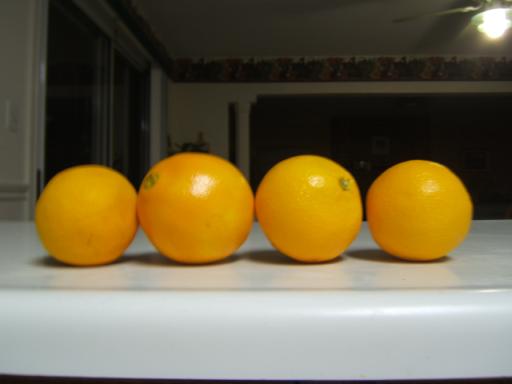The image is a detailed close-up of four oranges placed on a white countertop. The countertop appears to be a plain white melamine surface, reminiscent of the style popular in the 70s. The oranges are varying in size, with the two on the ends being smaller and the two in the middle being larger; the largest orange is second from the left. Each orange has a shiny, light orange skin with noticeable peel texture and small, green or brown stem ends. Behind the oranges, the background features a dimly lit living room setting, with a sliding glass door on the left and a large window straight ahead. The upper part of the walls is accented with a wallpaper border meeting the ceiling, and a ceiling fan with a light turned on is visible in the upper right corner. There seems to be a long white curtain hanging over the sliding glass door. Shadows cast by the ceiling light highlight the oranges, which are the primary focus of the image, though the focus is slightly sharper on the countertop's front edge.